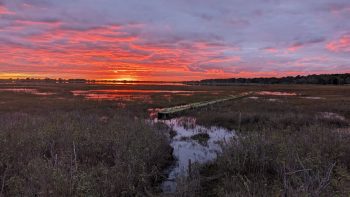This small, low-resolution outdoor photograph, measuring roughly two inches wide by an inch high, captures a mesmerizing sunset over a tranquil marshland. The upper half of the image is dominated by a stunning, vibrant sky where grayish-blue clouds merge with orange and red hues toward the horizon, eventually breaking off into smaller clouds. The glowing yellow sun is just below the horizon, painting the sky with warm, glowing tones. Below the horizon line, particularly on the left, we see a serene water system, part of a marsh or swamp, edged by long, unkempt reeds and tall grasses that appear grayish in the shadowed light. A very long, low pier or walkway extends from the right-hand side toward the center of the image, seemingly floating above the still water. Descending from the left side and down to the bottom, the marshy water and grass create a natural, wild beauty, while a lush, hillside forest is visible to the right, further enriching the landscape's depth and tranquility. No people are present, allowing the pristine natural elements to take center stage.